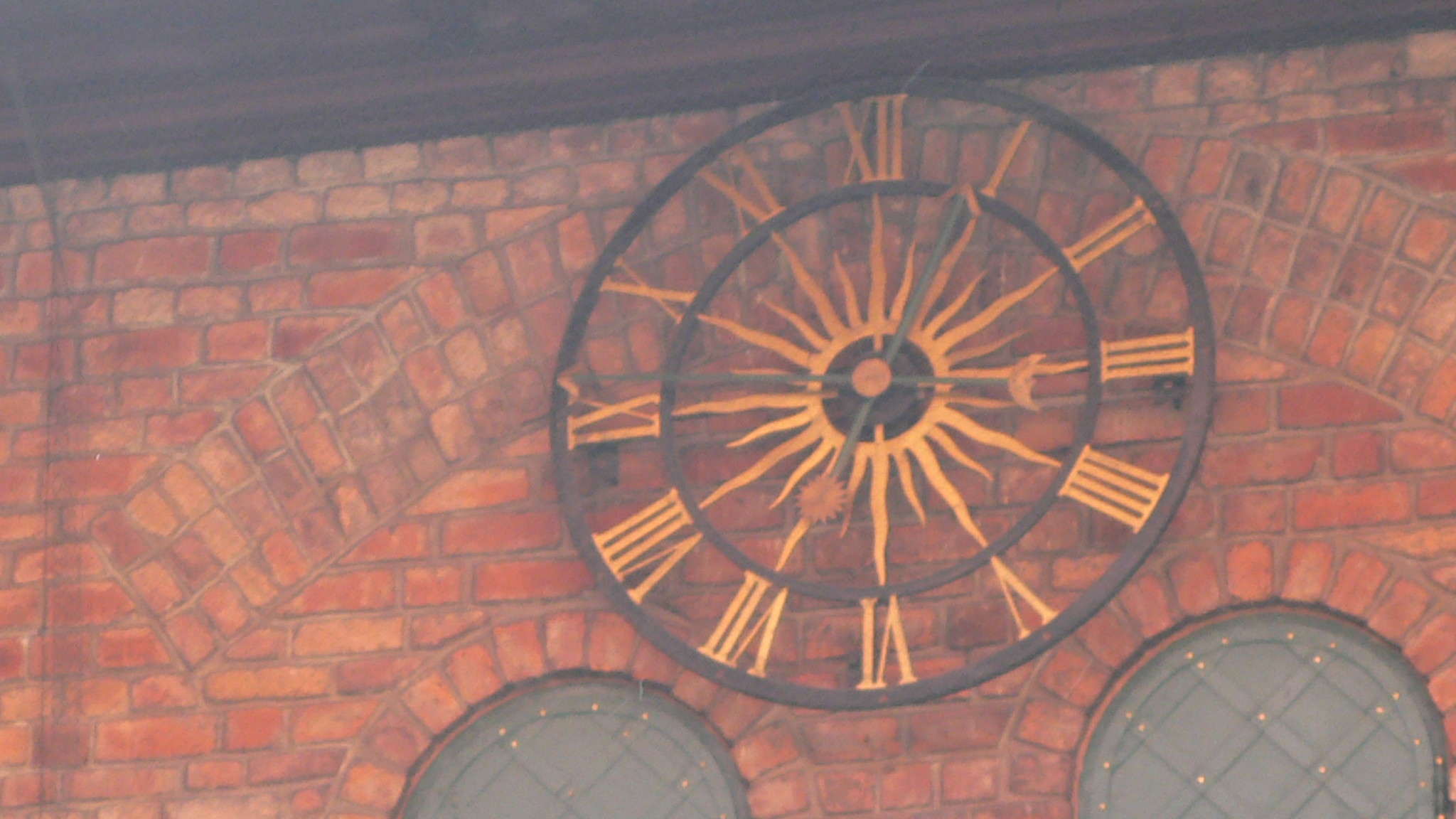This image depicts a detailed close-up of a striking exterior brick wall under construction, featuring a large, ornate metal clock as its centerpiece. The wall consists of reddish, rusty-colored bricks arranged mostly horizontally, with arches made of vertical bricks creating a rainbow-like frame around the clock. These arches sit above two partially visible circular glass windows. 

The clock itself is a commanding presence with an intricate design. It features a central golden sunburst pattern, with metallic rays emanating from the center, forming the clock's face. The outer and inner circles of the clock are dark gray or black, contrasting with the brass or copper-colored Roman numerals that mark the hours. These Roman numerals are set within a see-through mesh-like design in the metallic structure, giving the clock an airy, intricate appearance. The clock's hands are dark in color, and it is approximately 12:45, with the minute hand pointing to the 9 and the hour hand nearing the 1.